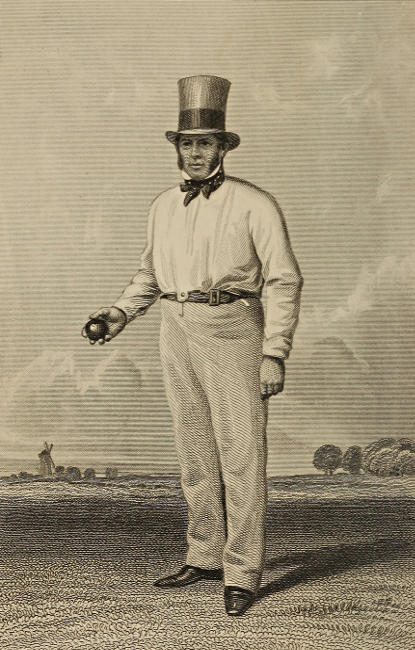This is a black and white engraving-style picture, possibly a sketch, depicting an older man with prominent mutton chop facial hair. He stands in a field characterized by texture markings, with a horizon that includes a small grey windmill on the left, smudges of trees in the center, and four larger, bushier trees to the right. Clouds with white outlines arc across a wispy grey sky above him. The man is dressed in light grey slacks with a dark belt and pointed black dress shoes. His white dress shirt, long-sleeved and buttoned up, is accentuated by a handkerchief around his neck. He wears a tall top hat, light grey with a black stripe just above the brim, giving it a distinctive dual-color appearance. In his right hand, he holds a dark ball and casts a shadow back and to the right. The picture exhibits lined patterns throughout, likely due to its age, adding a unique texture to the overall scene.